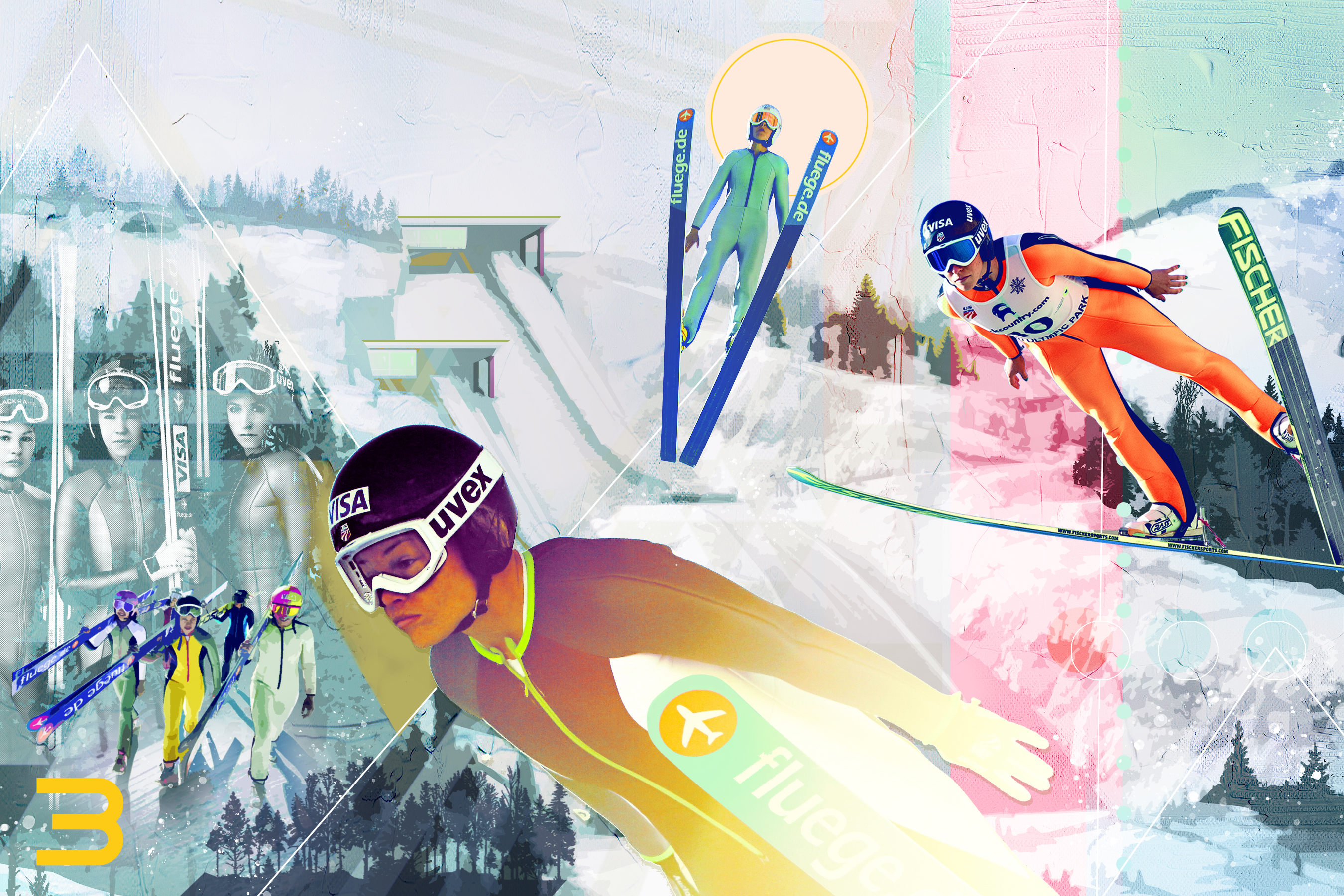The image is a vibrant collage of various snowboarding and skiing scenes, likely intended for an advertisement or a website. Dominating the left side, a black and white photograph showcases three skiers, their goggles up, posing with skis against a backdrop of snowy mountains. Below this, another trio of skiers carries brightly colored skis and helmets, standing out vividly against the overall teal background interspersed with a thick, slightly transparent pink stripe running towards the right. Prominently, there's a yellow, slightly pixelated number three on the bottom left.

At the center, a skier, leaning towards the left, sports a black and white helmet and a distinctive lime green and white outfit with a visible logo on the side. Moving towards the right quadrant of the collage, we see another skier with skis splayed apart, clad in an orange outfit with a white shirt overlay, marked by a helmet inscribed with the name "Risa."

Additionally, an almost horizontal, overexposed image of a woman skiing is suffused with purple and yellow hues towards the bottom. Finally, a depiction of the sun and snow-covered hills populates the background, blending seamlessly with the lively arrangement of athletes and their dynamic poses.